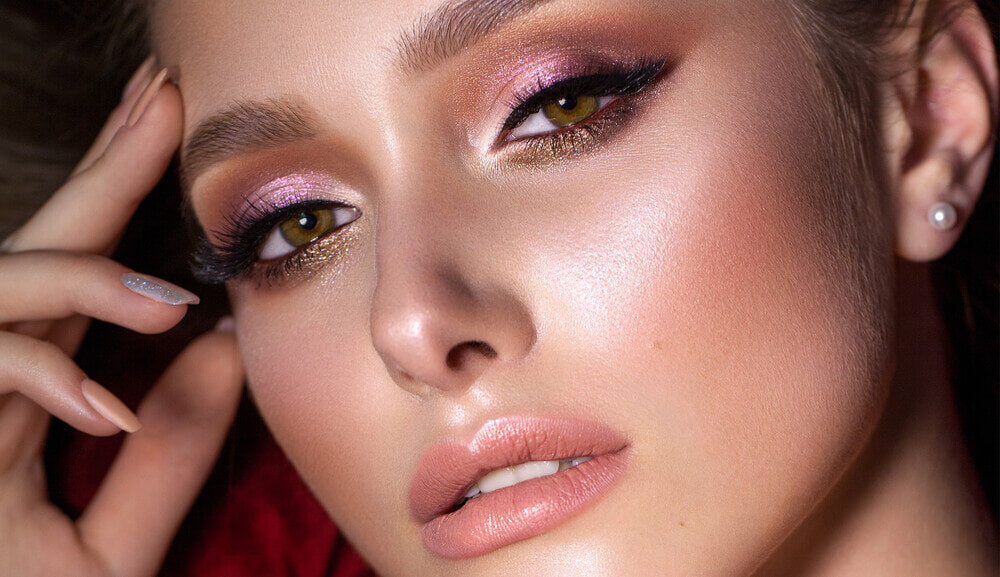This close-up glamour shot features a Caucasian woman, likely in a magazine beauty ad, showcasing her full face from her eyebrows to her chin, with her head tilted slightly to the left. Her brunette hair frames her face, revealing one ear adorned with a small pearl earring. Her expression is subtly seductive, with her slightly open mouth displaying her white, straight front teeth.

She's wearing heavy makeup: her eyes, which might be hazel or greenish-brown, are accentuated with well-manicured eyebrows, long false eyelashes, and a combination of metallic-brown and pink eyeshadows. There’s bronze eyeshadow and brown eyeliner beneath her eyes. Her upper lids are defined with eyeliner. Her complexion is flawless, featuring well-applied foundation and rosy cheeks. Her lips are coated in a peach-colored lipstick. 

Her manicured nails sport a peach base with sparkling pink and blue glitter accents. Her hand is gracefully posed against her face, adding to the overall allure of the shot.